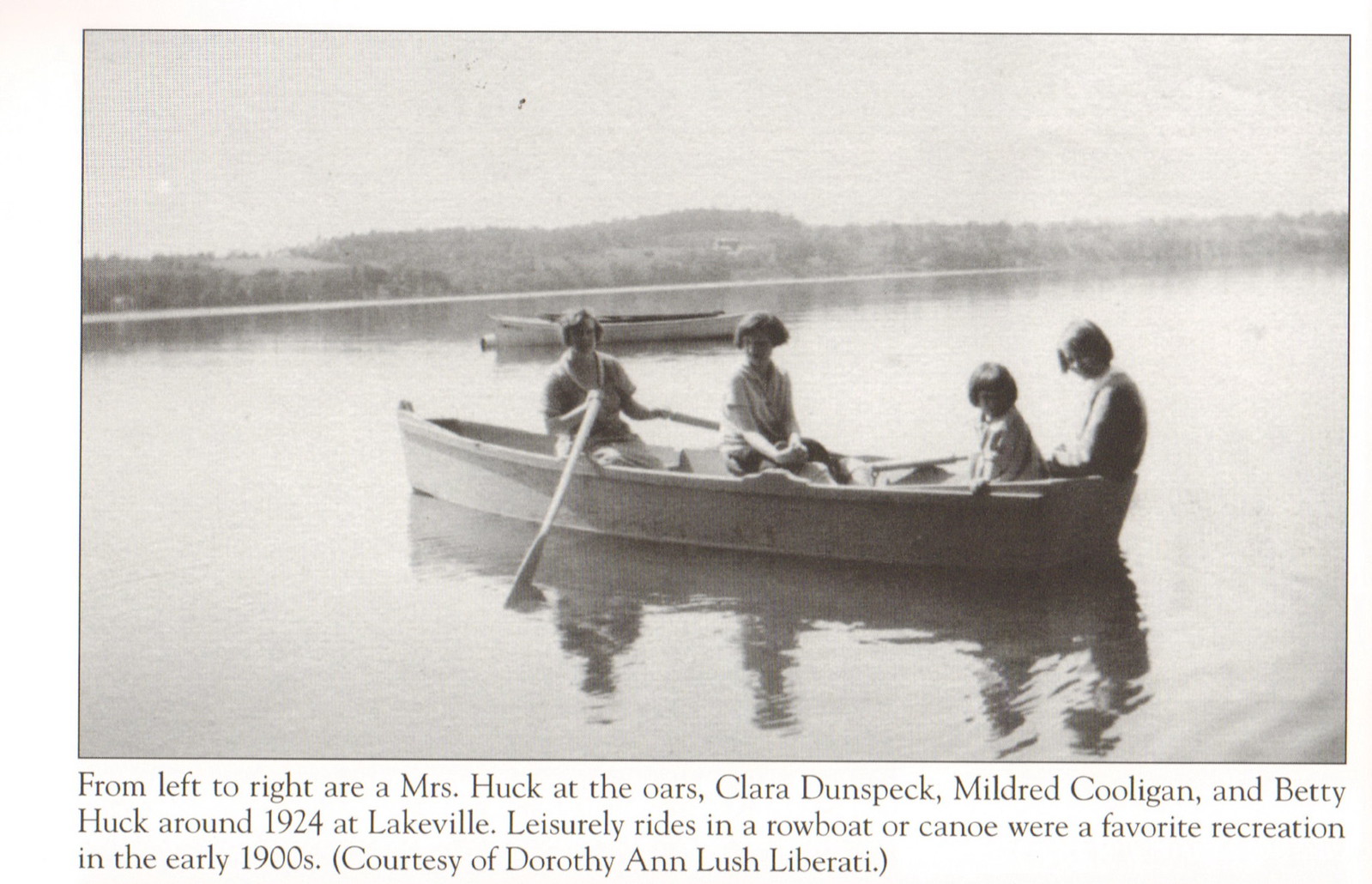This old black-and-white photograph, which appears to be a close-up scan from a newspaper, captures a serene moment of leisure from around 1924 at Lakeville. The image features an adult woman, Mrs. Huck, at the oars of a rowboat, accompanied by three young girls: Clara Dunspeck, Mildred Cooligan, and Betty Huck. They are situated in a calm lake, their reflections slightly visible on the water's surface. The backdrop includes an empty canoe and distant hilly terrain dotted with trees, suggesting a peaceful, possibly cloudy day. The caption beneath the photo notes, "From left to right are Mrs. Huck at the oars, Clara Dunspeck, Mildred Cooligan, and Betty Huck, around 1924 at Lakeville." It also mentions that leisurely rides in a rowboat or canoe were a cherished pastime in the early 1900s. The photo is credited to Dorothy Ann Lush Liberati.